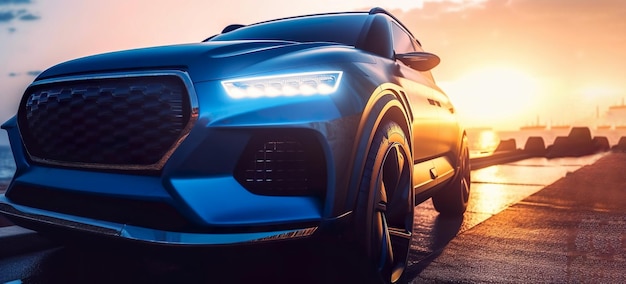The image showcases a close-up of the front grill and headlights of a dark blue car, set at an angle that highlights the left side front grill and part of the left side of the car. The elongated, horizontal headlights are shining, and the grill features a distinctive mesh design. The car is parked on a gray road under a sky that transitions from orange on the right to pink on the left, suggesting the time is either sunrise or sunset. The bright sun is clearly visible, casting reflections off the side of the car, enhancing its appearance as if in a product advertisement. The background consists of a beige or sand-colored hue, with the gradient sky adding to the serene atmosphere of the scene.